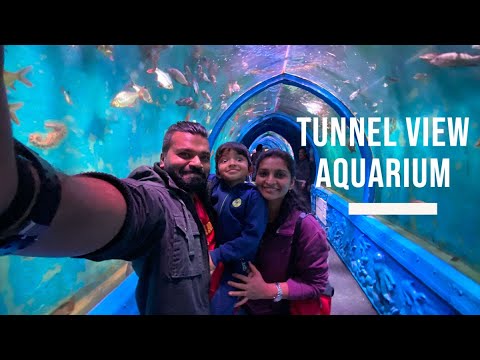The image depicts a happy family, likely of Indian or Middle Eastern descent, enjoying their visit to the Tunnel View Aquarium. They are standing within a unique see-through tunnel that runs through the aquarium, allowing visitors to be surrounded by blue-tinted water and a myriad of fish visible through the glass ceiling. The tunnel features short blue walls adorned with fish patterns and is supported by blue metal arches. In the foreground, a man on the left is taking a selfie with his family, comprising a woman on the right holding a cheerful young girl in the middle. The man is dressed in a gray jacket over a red shirt, the woman wears a purple top, and the little girl is wearing a blue outfit. The text "Tunnel View Aquarium" is visible on both sides of the tunnel, highlighting the aquarium's name. The family appears to be enjoying their time, captivated by the abundant aquatic life around them.